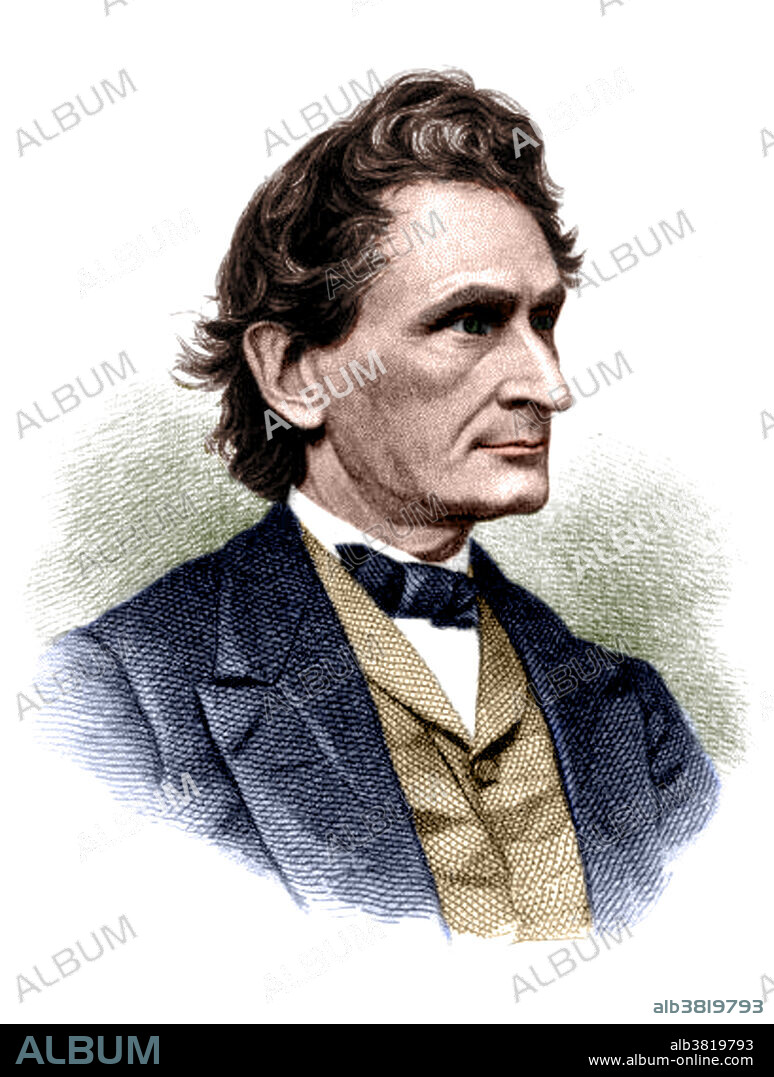This image features a sleek, white background with no borders on the left, right, or top sides. A thin black band runs horizontally along the bottom. On the left side of this band, 'ALBUM' is printed in blue against a black backdrop. To the right of this, in small white print, is the code 'ALB3819793,' beneath which the website 'www.album-online.com' is written.

Just above the black border, the code 'ALB3819793' appears again in blue print. Positioned above this text is the profile of a man, facing right. The image captures him from mid-chest upwards. He is dressed in a bluish-gray dress jacket over a light tan-colored vest, paired with a white button-up collared shirt and a matching bluish-gray bow tie.

The man, of Caucasian descent, features a straight aquiline nose with a subtle hook at the tip. His eyes are light-colored, framed by thick eyebrows and a pronounced brow. He has a thin mouth, a square jawline, and a large ear. His brown hair is curled and extends down to the nape of his neck. The background behind his neck and shoulders showcases a gradient, transitioning from a greenish tone to white.

Diagonally across the image, the word 'ALBUM' is repeatedly printed in gray, adding a dynamic visual element to the overall composition.